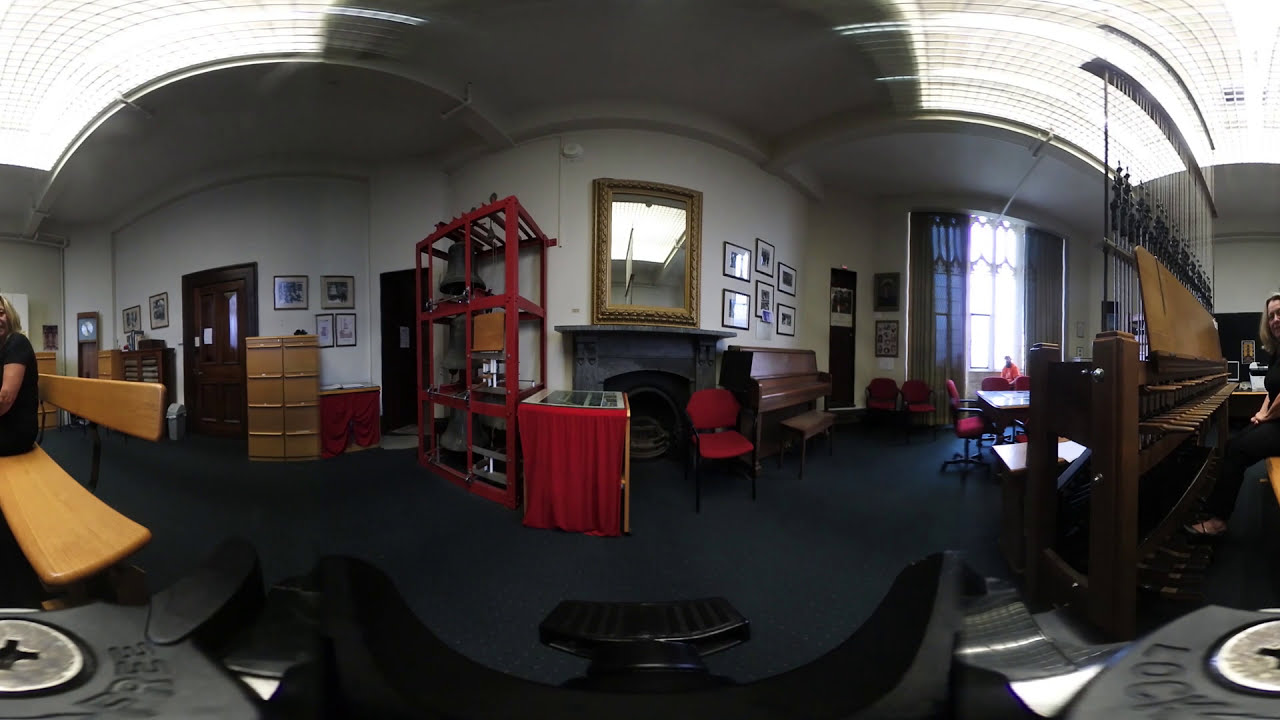This image depicts the detailed and eclectic interior of what appears to be an office or museum space, potentially the rectory of Notre Dame. The walls are painted white, contributing to the room's airy feel, which is enhanced by high, arched ceilings. In the center of the image, the focal point appears to be a large, open shelf laden with various items, notably including a heavy metallic bell on the third level. 

On the left side of the room are several notable features: a prominent brown wooden door with glass in the center, providing a sense of grandeur. Adjacent to this door, there is additional shelving and file cabinets, which further contribute to the room's sense of organization and function. Above these is a display of pictures and art, although they are angled and thus not fully visible. 

Continuing to the right, a grand fireplace with a black mantle dominates the wall, crowned by an ornate mirror that reflects parts of the room. An intricate red metal-framed display showcasing old bells adds to the antique and scholarly atmosphere. To the left of the fireplace sits a dark wood piano with a bench, and above it, more framed pictures and art adorn the wall. A red chair is positioned to the left of the piano, suggesting a space for casual sitting or waiting.

On the far right of the image, a large window invites in natural light, and in front of it, a blonde woman in dark clothing is seated on a bench. She appears contemplative, positioned next to a very old wooden instrument with rows of pedals and strings, indicative of its antique nature.

Additional features include various pieces of furniture such as tables or consoles and a grandfather clock, enhancing the room's historical feel. The floor is a dark color, providing contrast to the white walls. Overall, the room's arrangement and collection of items suggest it might be part of a historic office, museum, or ecclesiastical setting, rich with artifacts and character.